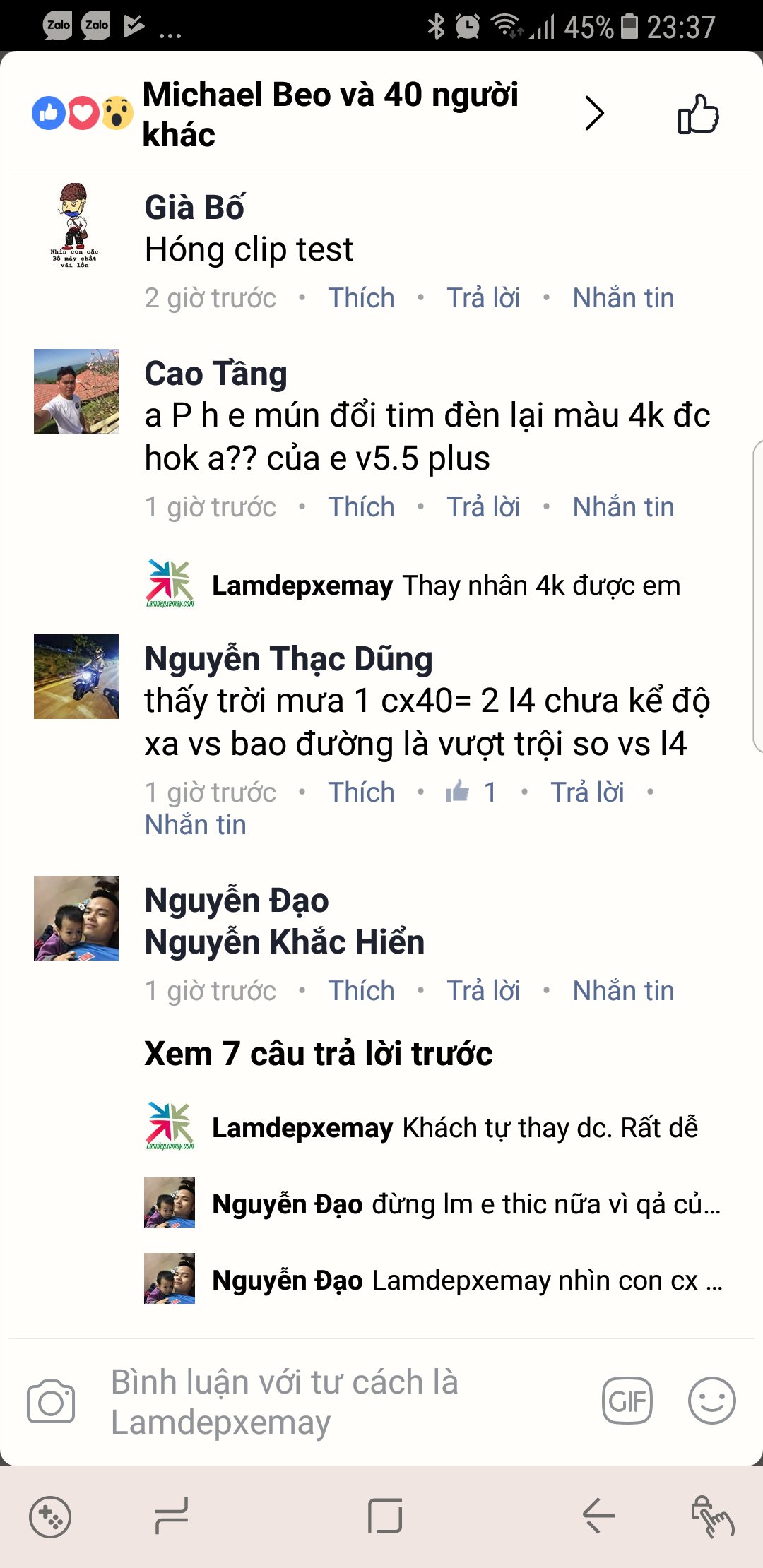This image is a detailed screenshot from an Android device, likely a Samsung phone, displaying a section of a Facebook conversation in Vietnamese. The interface reflects typical Facebook features, such as reaction options including thumbs up, heart, and surprise face. The conversation suggests a group text setting with names like Gia Bo, Sau Tang, and Nguyen Thac Dung highlighting its Vietnamese context. At the top of the screen, the status bar shows phone vitals: it’s 11:37 PM, the battery is at 45%, and both Wi-Fi and Bluetooth are activated. The bottom bar typical of Android devices includes symbols for navigation such as a circular home button, a square recent apps button, an arrow back button, and possibly a microphone or voice assistant symbol, emphasizing its identification as a Samsung device.